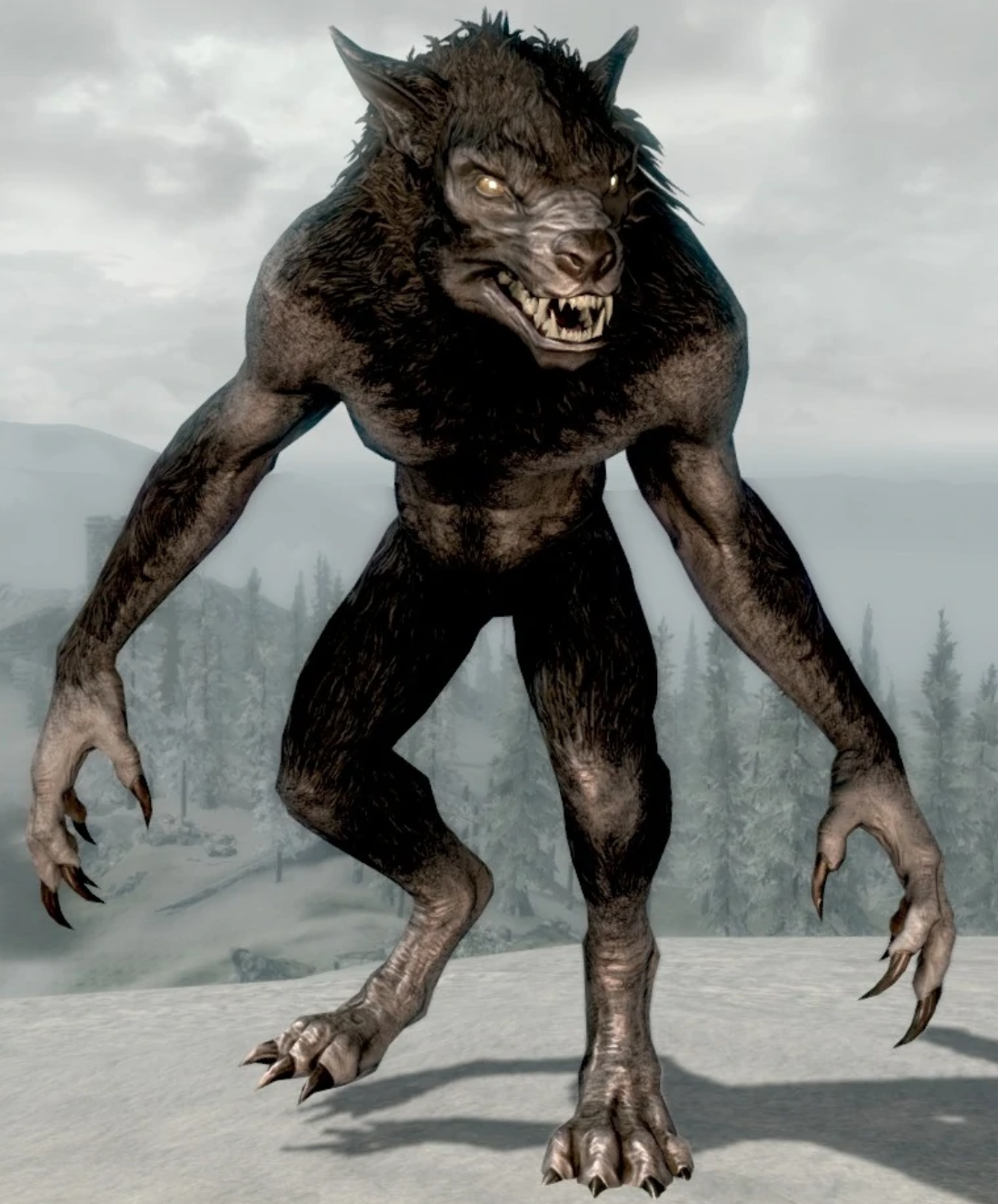A haunting, monochromatic illustration evokes the essence of a horror movie set in a foggy, winter landscape. The sky is an ominous shade of gray, filled with darker clouds that loom over a series of snow-covered mountains and densely packed pine trees. Emerging from this eerie backdrop is a towering, menacing werewolf with yellow, glowing eyes that pierce through the dim light. Its head, resembling that of an exaggerated wolf, is mostly black and brown with tufts of unkempt, dark hair. The creature's facial features include a prominent, black nose and a gray area above it, with its mouth wide open, revealing sharp, hulking fangs. 

The werewolf's build is muscular and imposing, with a bulked-up upper body and long, clawed arms that nearly touch the ground. Its torso is dark and bare, emphasizing its wild and feral nature, while its legs end in clawed feet, one of which is slightly lifted as though it's poised to lunge forward. An air of hostility radiates from its contorted, angry expression. 

Behind the beast, the scene is further heightened by the presence of a fortress-like brick structure that looms in the background, reminiscent of the Great Wall of China, adding to the unsettling atmosphere. Snow blankets the earth and the trees, and thick fog weaves among the mountains and pines, completing the chilling, wintry tableau.